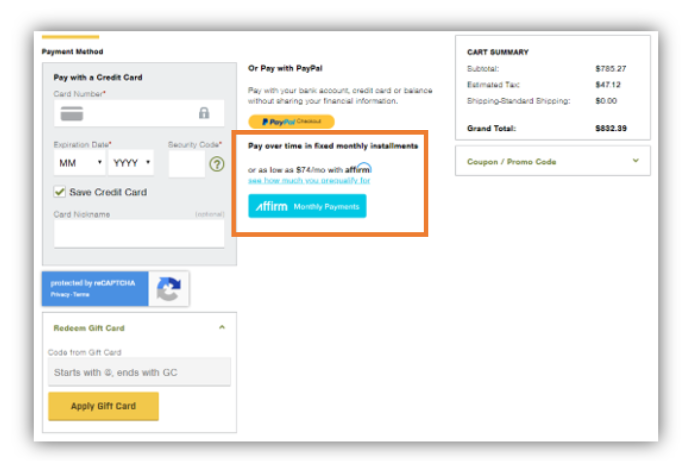The image depicts a highly blurred checkout page with various payment methods and summary details. The primary section shows options to pay with a credit card, presenting fields for card number, expiration date, and security code—all of which are blank. A "save credit card" option is checked despite the absence of any entered card information. A reCAPTCHA field has been completed successfully.

Additionally, there is an option to pay via PayPal, alongside a prominently highlighted option to pay overtime in fixed monthly installments, with a minimum of $74 per month using Affirm. Adjacent to the payment methods, a summary of the order is presented, detailing a subtotal of $785.27, estimated tax of $47.12, and $0 for standard shipping, culminating in a grand total of $832.89. Options to apply a coupon code or redeem a gift card are shown but remain unopened and unselected.

Despite the image's extreme blurriness and compression, making it difficult to discern specific details, it appears to serve as an infographic illustrating monthly installment payment options. There is no information on the items being purchased in the screenshot.